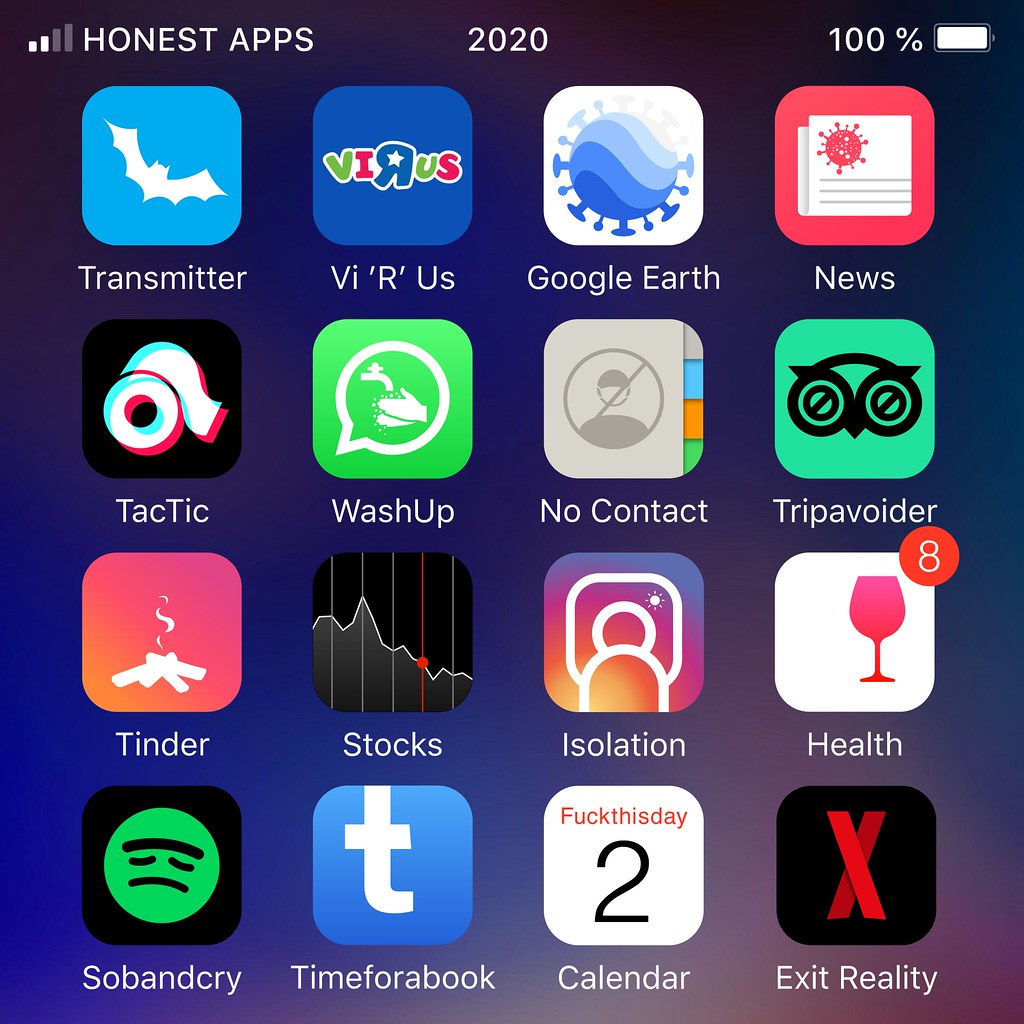In the satirical mock-up image titled "Honest Apps 2020" with a 100% battery, various parody app icons humorously reflect the realities of the year. At the top, a blue app named "Transmitter" mimics Twitter, featuring a bat logo. Nearby, a toy-store parody called "Vi R Us" evokes the iconic Toys R Us, while a corrupted Google Earth app, represented by a coronavirus symbol, sits beside it. The News app, ominously marked with a red coronavirus in the corner, indicates the pervasive nature of pandemic headlines.

"Tic Tac," a playful reimagining of TikTok, is symbolized by a roll of toilet paper, underscoring shortages. "Wash Up," an adaptation of WhatsApp, displays an icon of handwashing, promoting hygiene. The "No Contact" app, signified by a crossed-out human figure, highlights social distancing. "Trip Avoider" parodies Trip Advisor with an owl icon, dissuading travel. Meanwhile, "Tinder" retains its fiery symbolism, possibly hinting at the volatility of dating during these times.

The "Stocks" app shows a downward trend, reflecting economic concerns. "Isolation" replaces Instagram, indicating social separation. The "Health" app humorously features a wine glass rather than a medical symbol, alluding to coping mechanisms. "Sob and Cry," a take on Spotify, uses a frown-faced icon, capturing the year's general sentiment. "Time for a Book" humorously takes the place of Facebook, implying a shift to traditional pastimes. The Calendar app bluntly states, "Fuck This Day Too," encapsulating widespread frustration. Lastly, "Exit Reality," formerly Netflix, invites escapism, represented by an X symbol.